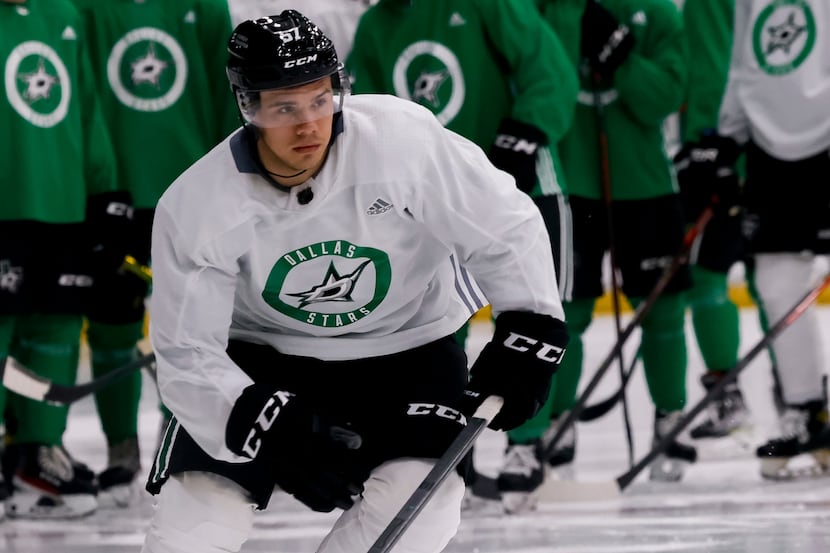The image captures a dynamic scene from an ice hockey game, featuring a central player from the Dallas Stars. The main player is prominently dressed in a white jersey emblazoned with a green circle that frames the words "Dallas Stars" in white, encapsulating a spiky star and a letter "D" at its center. He sports black CCM gloves, with the initials “CC” visible, and white padded pants beneath black shorts. His black helmet, which bears the number 57 and the CCM logo, includes a transparent visor. The player grips a black hockey stick with white tape wrapped around the top in his left hand while his right hand appears bent toward his knee, suggesting mid-motion engagement in the game.

In the background, several teammates stand on the ice, their heads cropped out of the frame. They share a mix of green and white jerseys, all adorned with the Dallas Stars circular logo, albeit the green-clad players feature a white logo. They wear black shorts with white stripes, similar to the central figure, and black skates with white laces. A yellow stripe is visible along the edge of the rink, encircling the players. The overall composition and detailed uniforms emphasize the central player's poised, action-ready stance, contributing to the compelling, competitive atmosphere of the photograph.